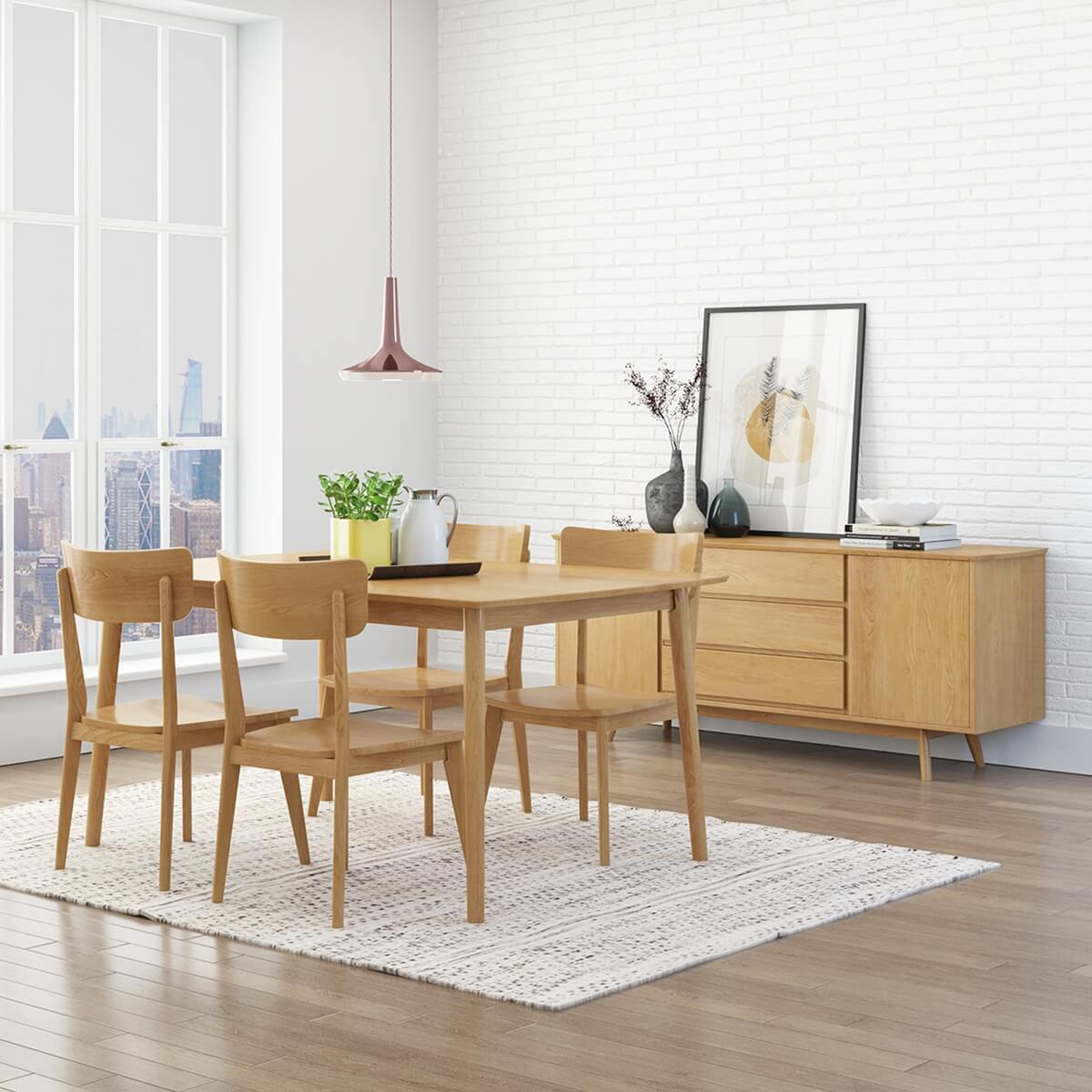The image depicts a modern, high-rise apartment, possibly located in a city like New York, as inferred from the visible skyline and skyscrapers outside the window. The room features a clean and contemporary design with a mix of white and wooden elements. A white brick wall contrasts with a solid white wall that includes a large window with an indentation, allowing a panoramic view outside.

In the center of the room, there is a white knitted rug upon which sits a wooden dining table surrounded by four matching wooden chairs, all in a rich brown color. The dining table is adorned with a small flower vase and a jug. A light fixture hangs above the table, illuminating the space warmly.

Against the white brick wall stands a wooden dresser. This piece of furniture hosts several decor items, including a small flower vase with purple blooms, a framed picture, and possibly other decorative components. The overall aesthetic is one of neatness and modernity, emphasizing the sleek, uncluttered arrangement of the furniture and decor.